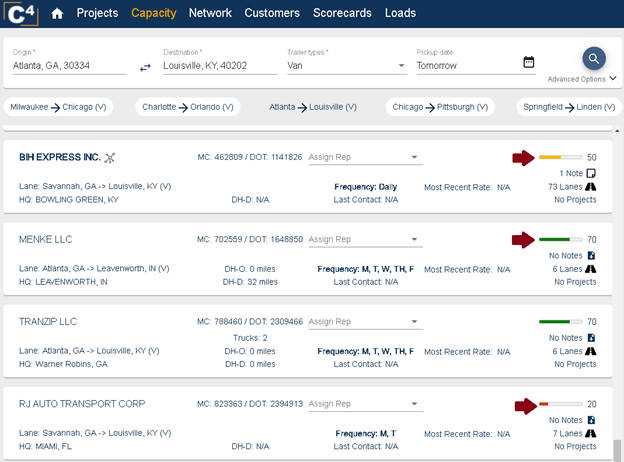**Screenshot of a Flight Information Website:**

The screenshot captures a detailed view of a flight information website. 

- **Header**: 
  - The header is positioned at the top of the page, characterized by a slim, dark blue bar with white text.
  - On the top left, there is a distinctive logo: a letter "C" followed by a superscript "4".
  - Adjacent to the logo, moving right, there is a white home icon followed by the word "Projects". Next, the words "Capacity", "Network", "Customers", "Scorecards", and "Loads" are displayed sequentially. The "Capacity" option is highlighted in orange, indicating it is selected.

- **Sub-header**:
  - Under the header is a medium grey background serving as a sub-header.
  - A white rectangle with text boxes and labels sits on top of this background.
  - The fields include:
    - **Origin**: Atlanta, Georgia, designated by the number "3334".
    - Two blue arrows, one pointing right and one left.
    - **Destination**: Louisville, Kentucky, designated by the number "4202".
    - **Trailer Types**: Denoted as "Van".
    - **Pickup Date**: Marked "Tomorrow", accompanied by a calendar icon.
    - A dark blue circle with a white magnifying glass icon signifies a search function.

- **Advanced Options**:
  - Beneath the white rectangle, there's a label "Advanced options" with a downward-pointing arrow.
  - Below this label, five selections are presented, each in a white rectangle with rounded edges except the central selection, which lacks a background.
    - The destinations listed are:
      - Kentucky (arrow pointing right)
      - Chicago (V)
      - Charlotte (Orlando, V)
      - Atlanta (Louisville, V) - This selection does not have a background.
      - Chicago (Pittsburgh, V)
      - Springfield (Linden, V).

- **Main Content**:
  - The main body of the website features multiple lines on a white background, each line showcasing different destination combinations.

This breakdown provides a comprehensive guide, emphasizing the structure and various elements that make up the flight information website interface.